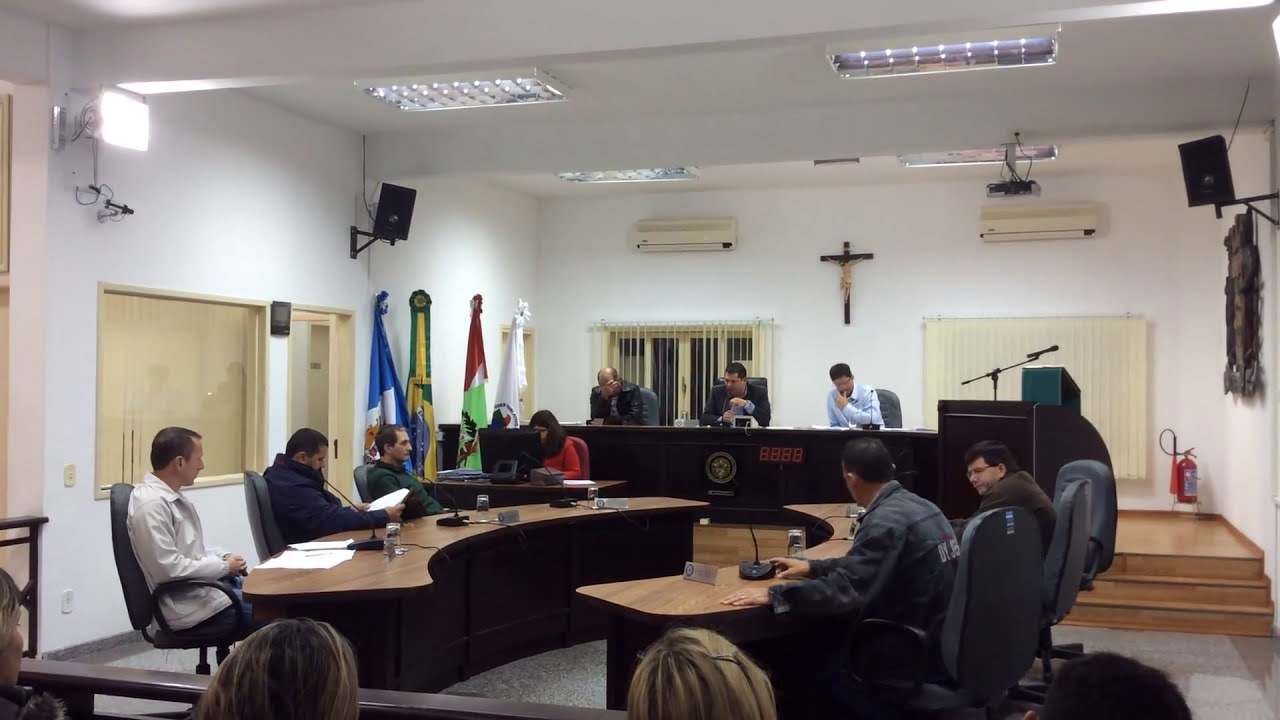The photograph depicts the interior of an official, brightly lit room with whitewashed walls, most likely inside a church or courtroom setting. The room features a white ceiling with fluorescent lighting. Centrally, on the back wall, there's a large crucifix. Below the crucifix, there's an elevated desk or podium with three men in official attire seated behind it, each equipped with a microphone. Flanking the main desk on either side are two curved tables facing each other; three men are seated at the left table while two men occupy the right. A woman in red, positioned near the left table, is seen typing behind a computer screen, presumably taking notes. The room also has visible air conditioners, loudspeakers located near the top of the walls, and a series of flags on the left side. At the bottom of the photograph, a wooden partition separates the main area from observers whose heads are visible, indicating their attendance at the meeting being conducted.